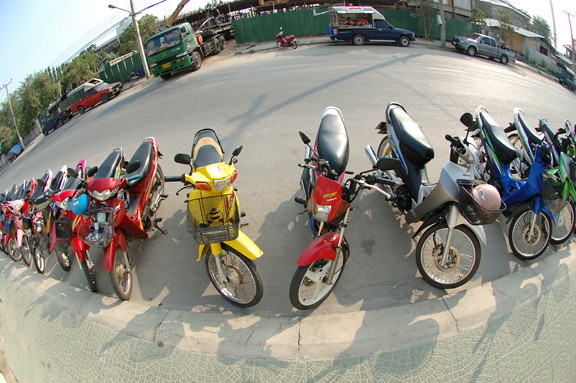In this color photograph taken with a fisheye lens, we see a dozen or more mopeds or city scooters lined up on a street, predominantly in red, yellow, and a few other colors like blue, green, silver, and black. Most of the scooters have black leather seats. The fisheye effect gives the image a distinctive curvature, making the central scooters, a red one and a yellow one, appear larger. Parked along the street behind the scooters are various vehicles including a green truck, a blue food truck, a silver utility truck, and a red pickup truck. Power lines are visible overhead, and there are trees and a green fence in the background. One individual is seated on one of the scooters, suggesting they may be available for rent. The overall setting hints at a European or Eastern European urban environment.